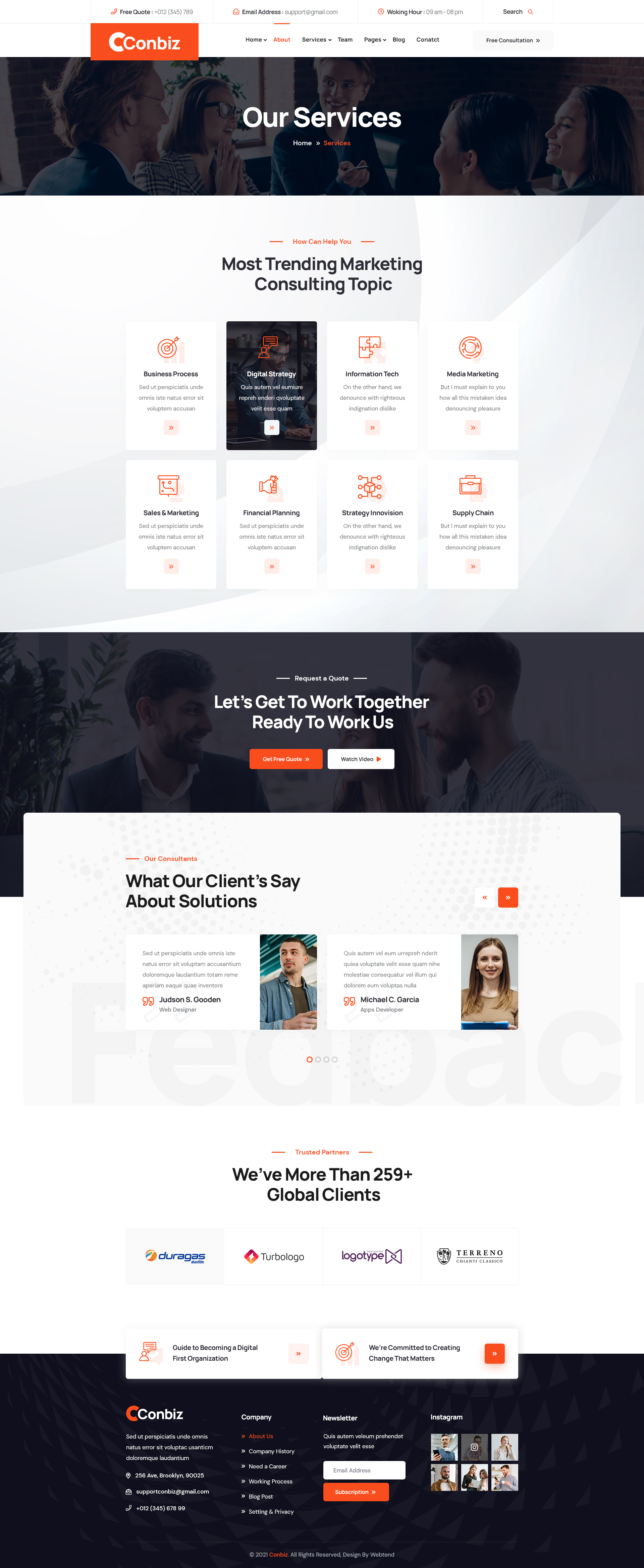This image showcases a webpage. At the top, there are three quotes followed by a contact number (012-345-789) and an email address (support.gmail.com). The working hours are listed as 9am-8pm. The website features the brand name "CONBEES" prominently. 

The navigation menu includes categories such as Home, About, Services, Theme, Pages, Blog, and Contact, along with a "Free Consultation" section. The main content highlights "Our Services" and lists several categories: Most Trending Marketing Consulting Topics, Business Process, Digital Strategy, Information Technology, Media Marketing, Sales & Marketing, Financial Planning, Strategic Innovation, and Supply Chain.

Additionally, there's a call-to-action section that reads "Let's get to work together" and "Ready to Work with Us?" Lastly, there's a testimonial section indicating that the company has more than 259 global clients with client reviews about their solutions.